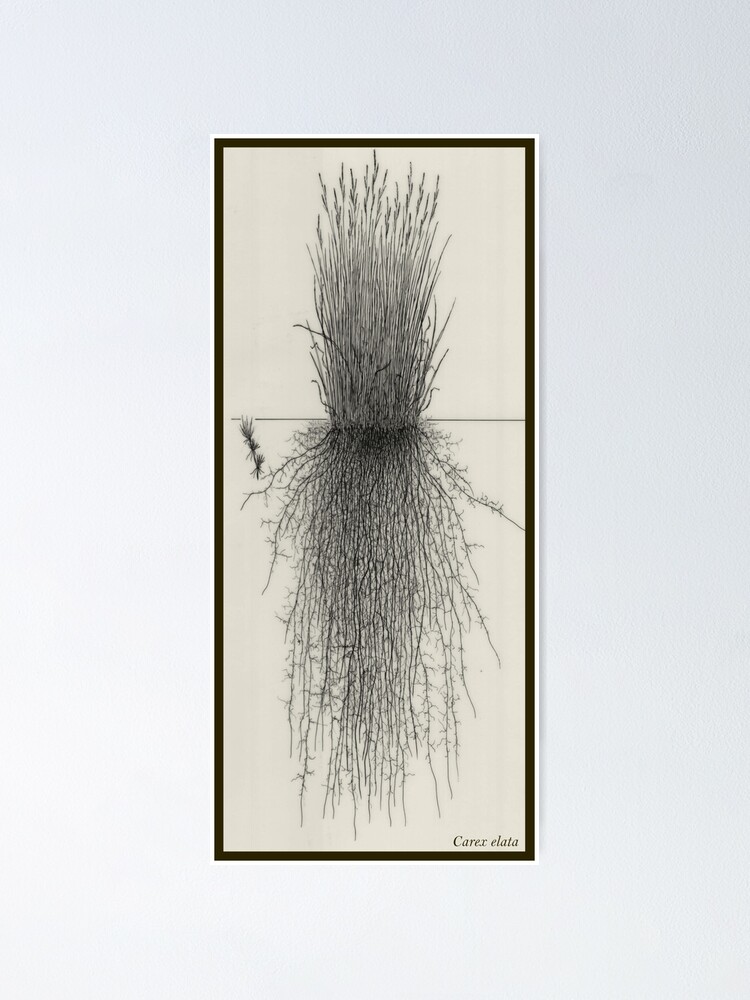The image displays a detailed black and white pen and ink botanical illustration, prominently featuring a tall clump of flowering grass. The artwork is visually divided by a horizontal line, approximately two-thirds of the way up, separating the above-ground foliage from an intricate depiction of the plant's underground root system. The roots are highlighted with hair-like structures and various sprouting details, emphasizing their complex nature. The drawing is signed by an artist whose name begins with a 'C,' located in the bottom right corner. The image itself is set against an off-white canvas with a thin white border, encapsulated within a thicker black frame. This framed artwork hangs against a light gray wall, adding a sophisticated contrast to its surroundings.